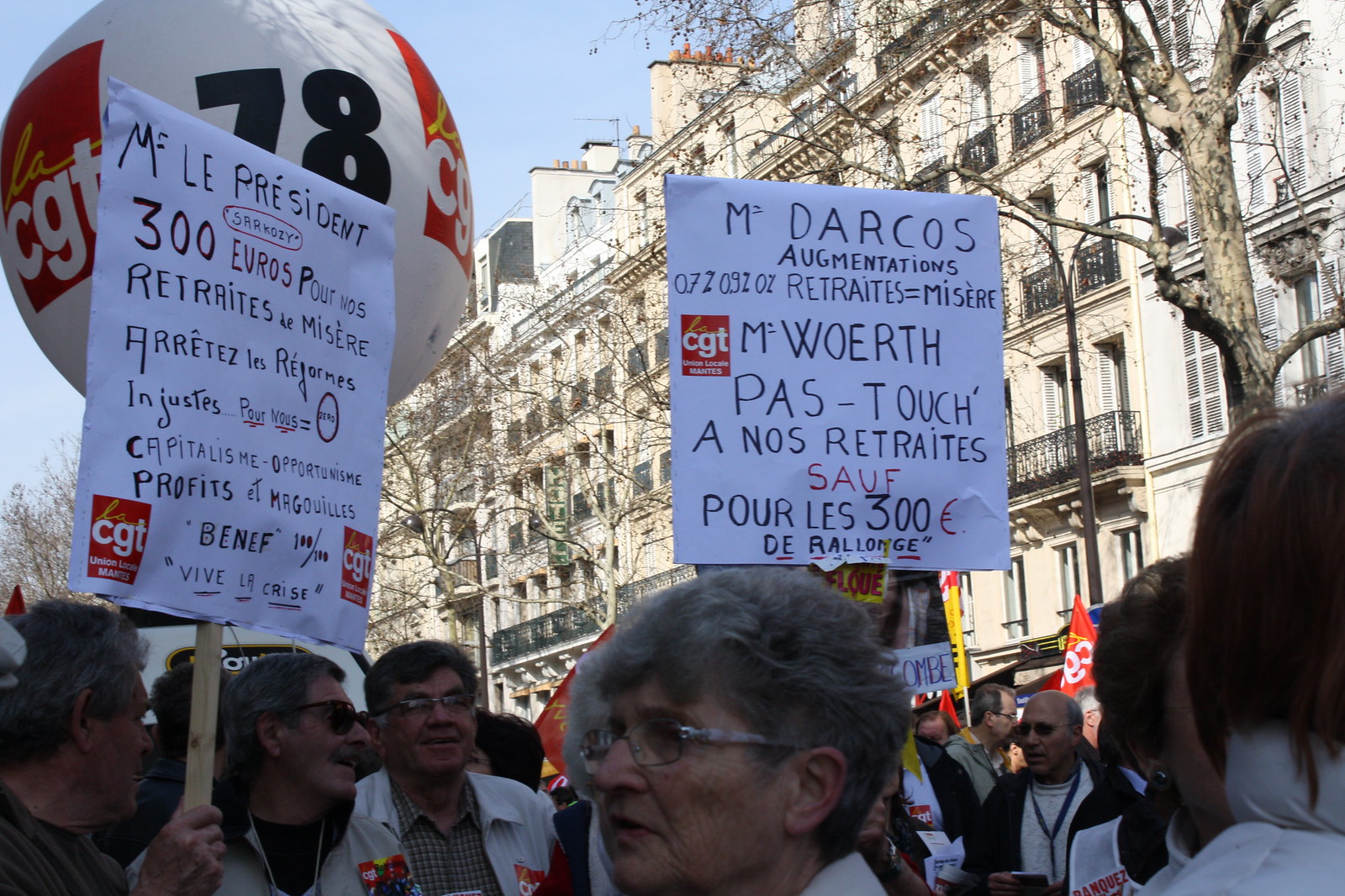This is a photograph of a French protest taking place in a European city with old, multi-story buildings in the background, featuring arched windows and balconies with black railings. The scene includes about ten people, with one person prominently ahead and others visible from the chest up. An older woman with gray and brown hair and glasses stands at the center bottom, surrounded mostly by men holding up handwritten signs on wooden sticks. The signs, written in French, include messages addressing "Ms. Le President," "300 Euros," "retirees," and "misery," indicating a protest about retirement age or benefits. Red stickers with white letters "CGT" are noticeable on some signs and a large white balloon with the number 78 and "CGT" in black hovers in the upper left. The atmosphere suggests a winter setting, with leafless trees in front of the buildings and a clear, blue sky.